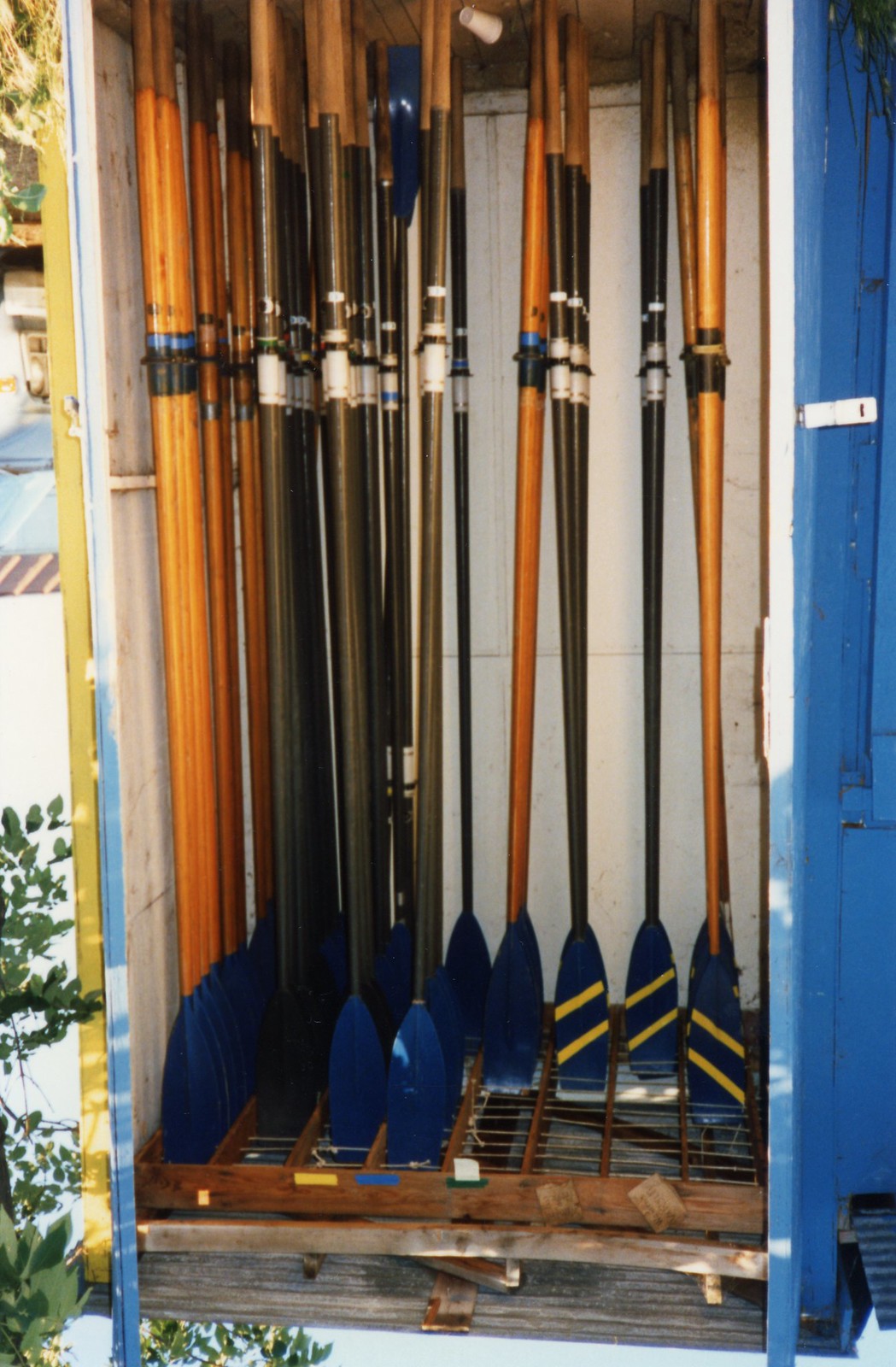The image depicts an outdoor scene showing an open blue metal storage cabinet, approximately the size of a phone booth, containing about 25 rowing oars. The cabinet's doors swing outward, revealing the neatly organized oars standing upright within a wooden bracketed grid meant to safely secure and prevent the oars from damaging each other. Each oar has a wooden handle, varying in color from medium brown to darker shades, with some appearing almost desaturated gray. The blades of the oars are uniformly navy blue, with several featuring angled yellow stripes. The cabinet is situated amid green foliage and trees, visible to the photograph's left side, suggesting it is placed outside on a paved surface.